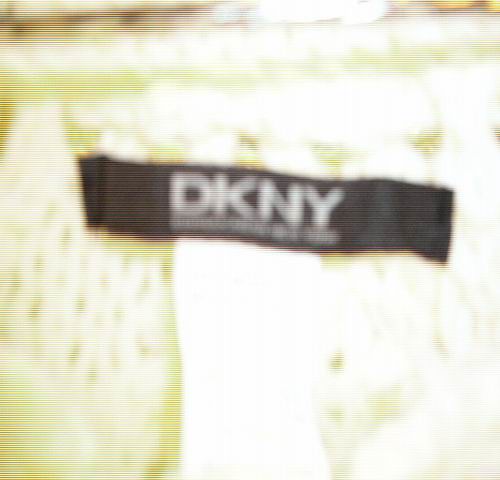This image shows a very blurry, close-up shot of a clothing tag. The tag, centrally positioned and rectangular in shape, is black with white lettering that reads "DKNY." Below the "DKNY," there is additional smaller text that is illegible due to the blurriness. The item of clothing the tag is attached to appears to have a shiny, textured material with a combination of light gold, almost yellow, and whitish-greenish colors. The fabric has vertical, striated lines running through it, giving it a somewhat holey appearance reminiscent of fish skin. Towards the top of the image, there is a darker, brownish shade, making the overall color scheme very mixed with white, light green, and light gold elements. The image is of a relatively small scale and features a clear, white strip running down the middle, separating the pattern. The focus is significantly out of focus, making finer details difficult to discern.